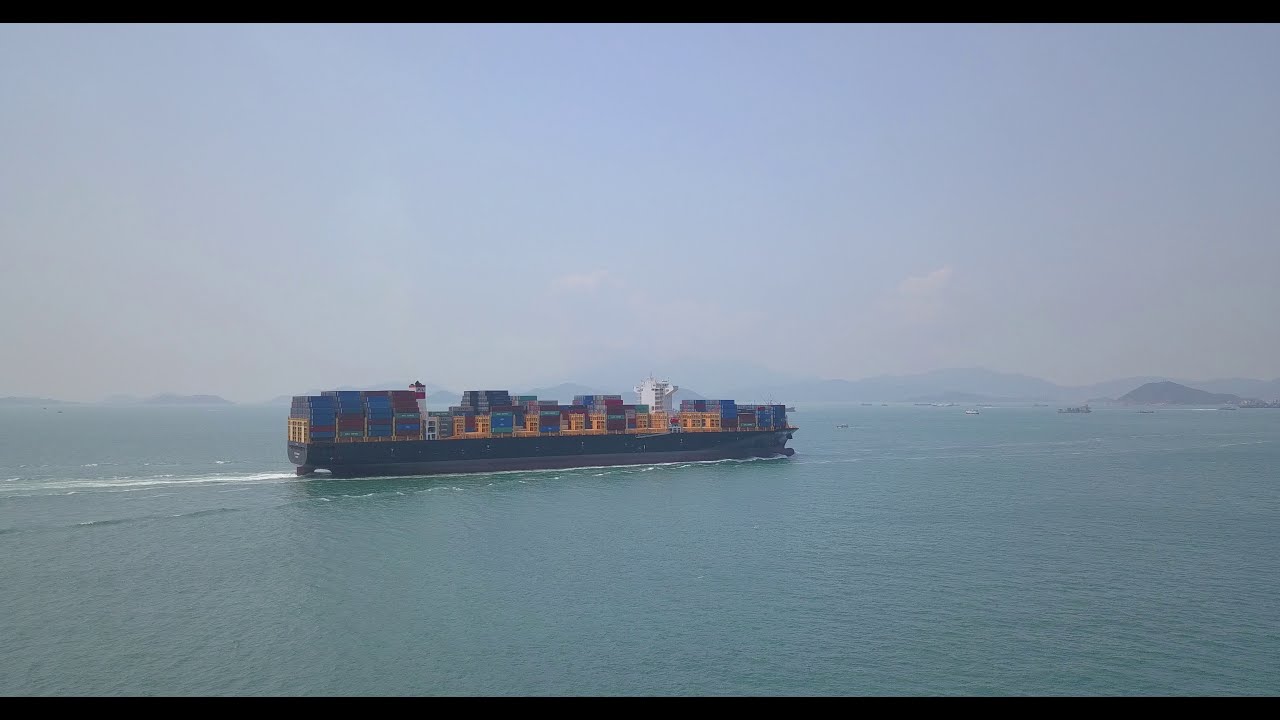In the image, a long cargo ship traverses a large, calm body of water, possibly an ocean or a big lake. The water is a deeper turquoise, and the ship leaves a trail of white waves behind it. The ship itself is predominantly navy blue with black and brown accents. On its deck, an assortment of vibrant shipping containers in yellow, blue, red, and green are neatly stacked. The deck also features a distinct white lookout tower. The sky above is hazy, transitioning from a light blue at the horizon to a deeper blue at the top. In the distance, faint outlines of hills and mountains linger behind the grayish haze, adding a serene backdrop to the scene. Smaller ships can be spotted on the water, contributing to the overall tranquility of the picturesque setting.